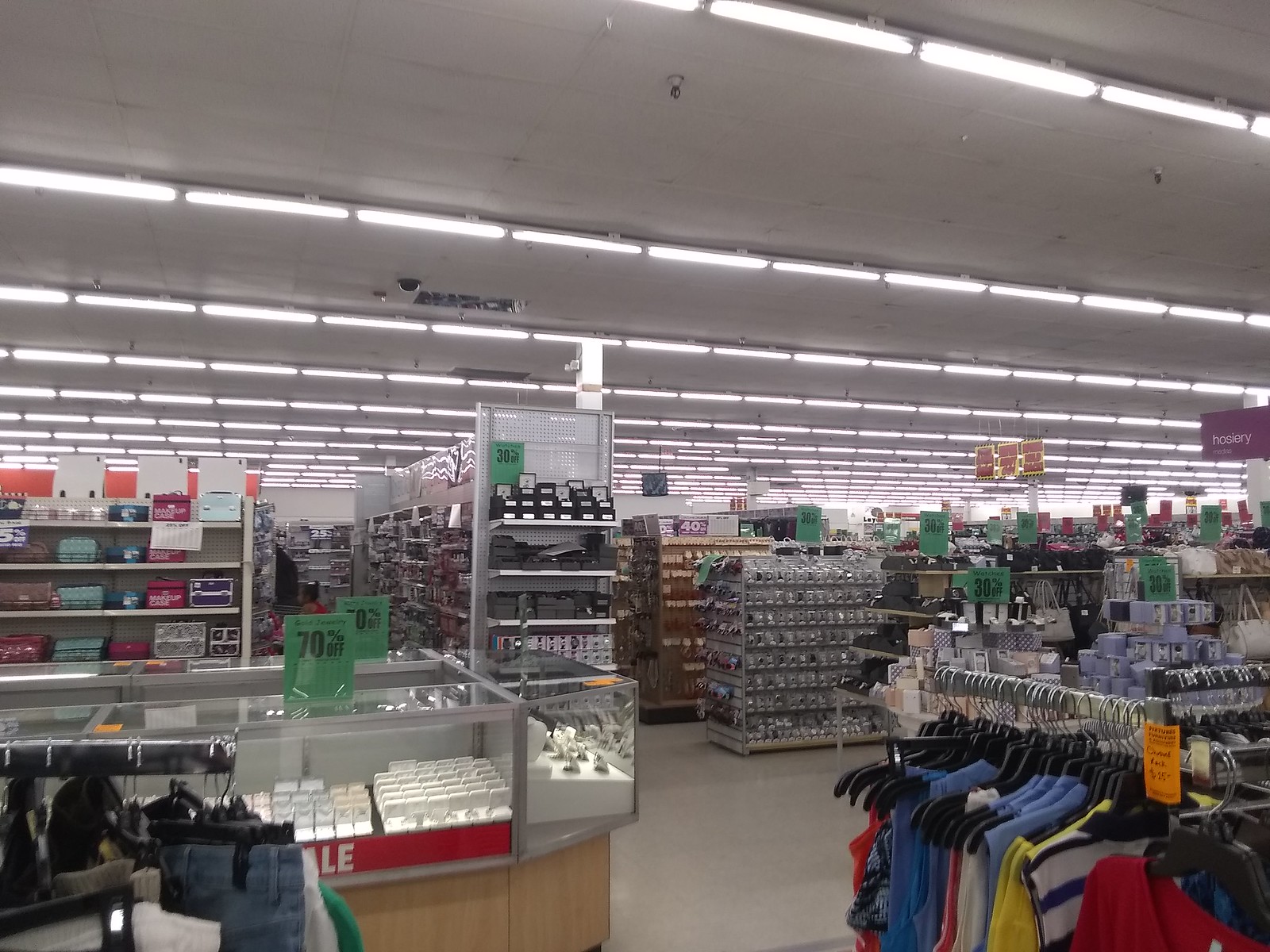The image, taken from a first-person perspective inside a department store, showcases a retail environment brimming with diverse merchandise. The store features a characteristic white, grid-style ceiling adorned with long fluorescent strip lights, security cameras, and sprinklers. Dominating the foreground are clothing racks: the bottom left rack holds pants, while the bottom right displays sleeveless shirts. The left side of the image also reveals a glass-encased jewelry counter with a prominent 70% off sale sign, indicating a major sale event, possibly a going-out-of-business sale, as suggested by various green and orange signs advertising discounts of 30% and more. In the midground, additional racks display items like purses, and further back, there are aisles dedicated to makeup, household items, and other gifts. A sign for hosiery is visible in purple, positioned above an aisle that houses watches and shoes. The entire store is brightly lit and cluttered with products and sale signs, creating a busy and bustling atmosphere.